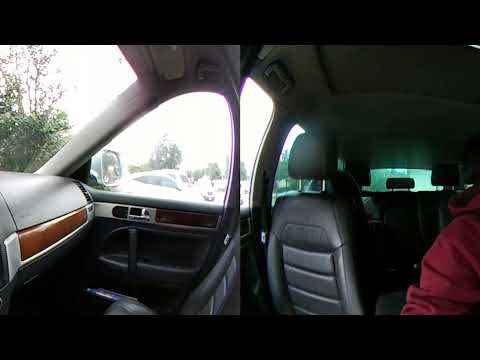The image is a composite of two photos showcasing the interior of a car from different angles. On the left side, we see the interior from the driver's perspective, focusing on the passenger seat, glove box area, door, and a window view revealing a parking lot with other vehicles. The bright sunlight outside makes it challenging to discern further details. The right side of the image shifts to an angle from the dashboard looking back, highlighting part of the passenger seat and the back of the vehicle. Here, we also catch a glimpse of the driver’s arm clad in a red jacket or hoodie. The interior of the car appears dark and sparsely decorated, with a plasticky dashboard and black seats. Out the rear window, faint outlines of trees and possibly a building are visible, though the brightness makes them difficult to see clearly.